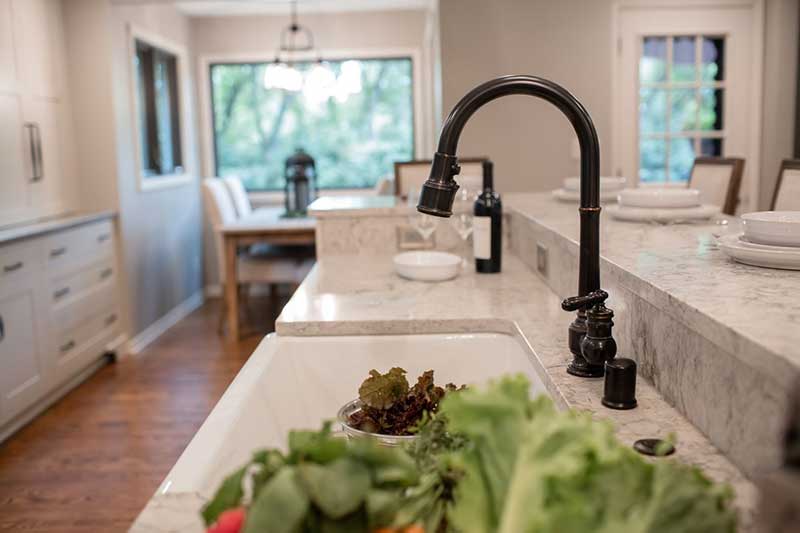This color photograph captures a close-up view of a modern kitchen centered around a white farmhouse sink embedded in a white and gray marble countertop. The black brushed brass faucet elegantly arches over the sink, accompanied by matching handles. Distinct groups of lettuce, including dark green, light green, and a mix of purple and dark green, are positioned on the countertop to the right. A bottle of wine with a white label and two empty wine glasses stand nearby, sharing the counter space with a small white ceramic bowl.

The kitchen features bright white cabinetry with numerous drawers to the left, a white door leading outside to the right, and a large window straight ahead offering a view of green tree branches. The upper level of the counter, functioning as a bar area, is set for dining with three white circular plates and bowls. Behind the kitchen, a blurred dining area with a light brown wooden table and four white chairs is visible, partially obscured by natural light filtering through another window overlooking leafy trees. The floor is light brown wood with dark brown splotches, complementing the white vase board.

Above the dining table, a chandelier with multiple lights hangs, illuminating the setting, while additional kitchen details like a black-framed picture and a small, indistinguishable circular device add depth to the scene. This kitchen captures both elegance and practicality, with thoughtfully placed items creating a cozy yet sophisticated atmosphere.